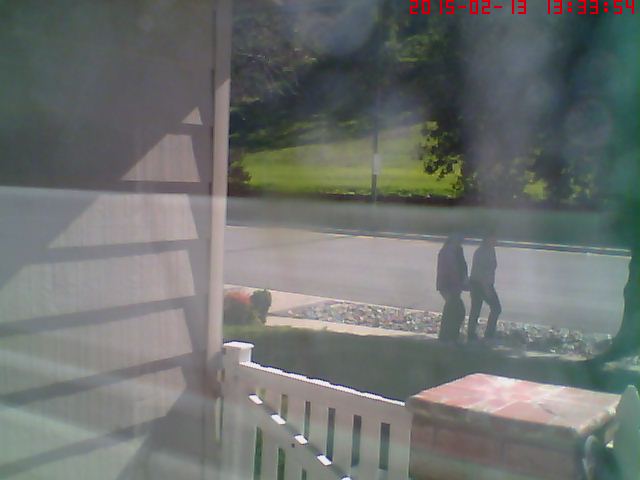This image, seemingly taken from a security camera inside a house on February 13th, 2015 at 13:33:54, has a hazy, filmed-over appearance as if viewed through a glass window or screen door, and features some visible reflections. Dominating the left side of the frame is a gray, wood-sided house with angled paneling, flanked by a white picket fence that leads to a small brick pillar. This fence continues along part of the scene. Beyond the white gate and brick structure, the scene opens up to a sidewalk and a strip of gravel along the curb by the road. There are two indistinct figures walking on the sidewalk, seemingly holding hands, moving from left to right. The street itself is bordered by a green lawn, several trees, a flower bush, and a green bush adding to the scenery. Farther in the background, a field with additional trees can be seen. All these elements together create a detailed snapshot of a quiet residential street from a porch view.